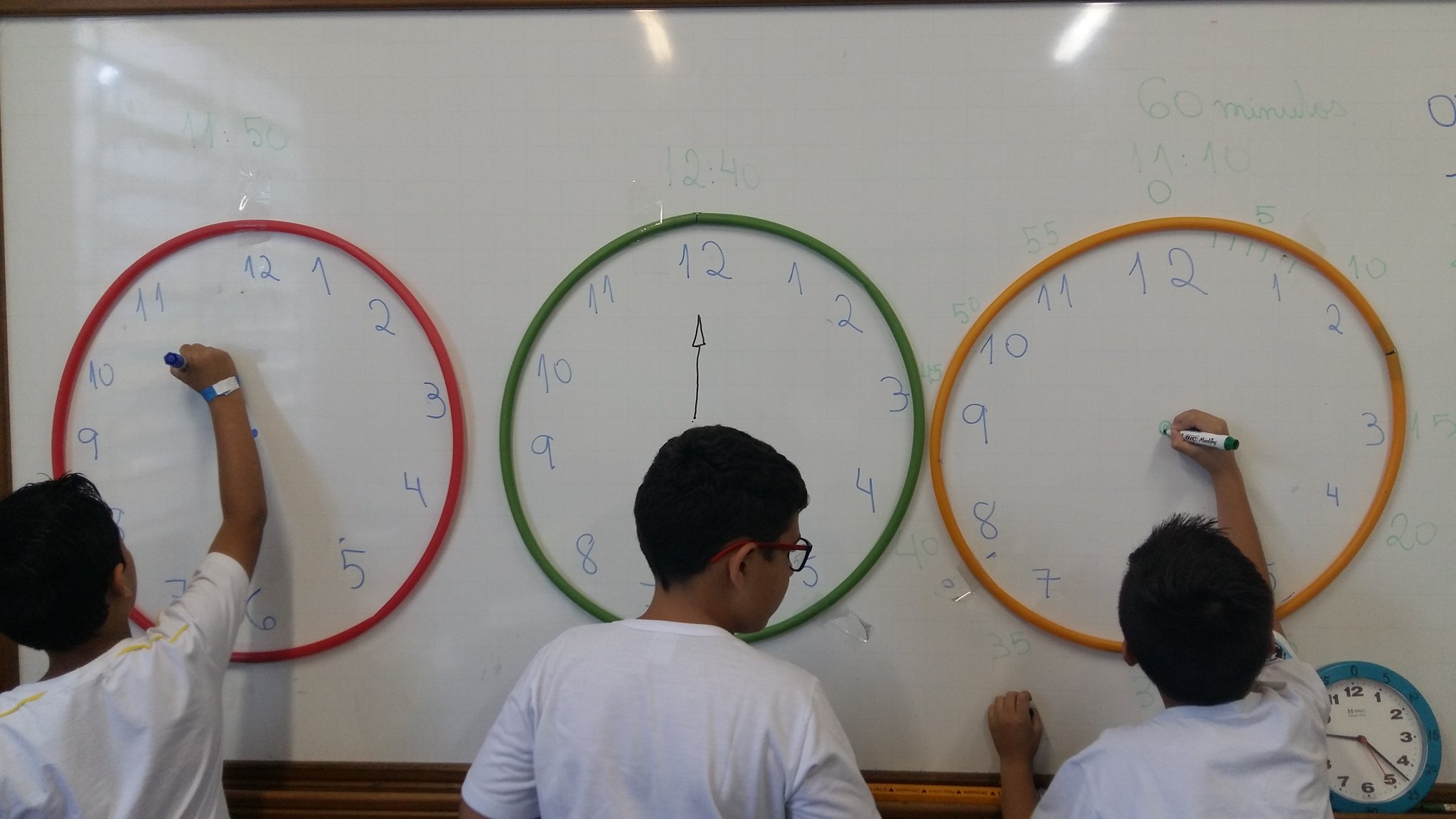Three students are standing at a large whiteboard, with their backs to the camera. The whiteboard is covered with a mix of marker and chalk writings. Brown circular mats, designed to look like clocks, are placed on the floor directly in front of the children. The students on the left and right are actively writing on the board with markers, each raising their arm to reach the surface. The middle student, distinguishable by their glasses, is glancing towards the student on the right, observing their actions. The scene captures the collaborative and interactive learning environment.